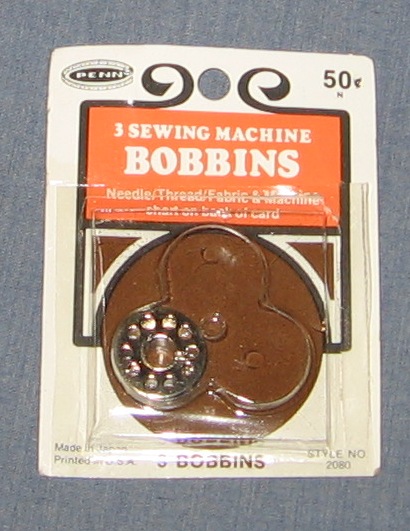This image depicts a vintage packaging for sewing machine bobbins. The package is designed with a white cardboard background and features a distinct blue fabric as the backdrop. At the top left corner, there is a brown oval spot with the brand name "Pin" displayed in white letters. The upper right corner clearly marks a price of 50 cents, suggesting its age. Central to the design is a prominent orange rectangle with white text that reads, "Three Sewing Machine Bobbins," providing the product description. Below this, there's an additional brown triangular section with further details. Despite indicating that the package should contain three bobbins, only one remains—a chrome, cylindrical piece with a circular pattern of holes, akin to a rotary phone dial, encased in a plastic mold. The design of the packaging, with its ability to hang on display racks, and the aesthetic elements, such as the text boxes and logo, display a nostalgic, vintage charm.